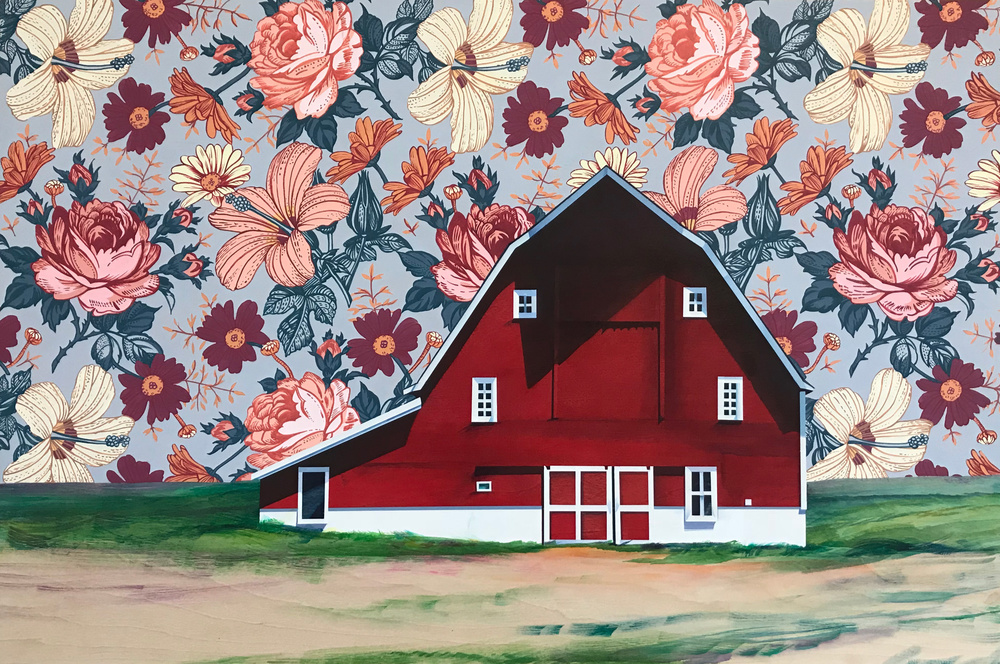The image is a detailed and vibrant artistic rendering that combines various materials and techniques to create a surreal yet cohesive scene. Dominated by a large red barn situated at the center, the structure features multiple stark white-trimmed details, including small windows and doors with paneled outlines. The barn is intricately designed with sharp contrasts: two windows under the pointed roof, additional windows below, and a large door at the base featuring six square panes, as well as a four-pane window on the right-hand side.

Surrounding the barn is a foreground of textured ground consisting of green grass interspersed with brown dirt and a sandy trail running horizontally in front. Adding to the complexity, the background substitutes a traditional sky with a rich collage of floral wallpaper. This backdrop showcases an array of flowers such as large pink peonies, pink daffodils with pronounced stamens, white and magenta daisies, chrysanthemums, and lilies. The flowers are depicted in shades of pinks, reds, oranges, and maroons, set against a light blue background, contributing to the dreamlike atmosphere of the piece. The interplay of naturalistic elements and stylized patterns emphasizes both depth and artistry, making the scene both intriguing and visually striking.